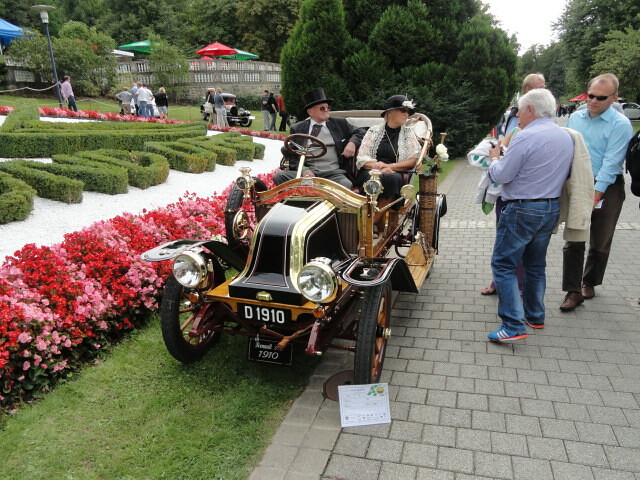In this captivating photograph, an exquisitely restored vintage automobile, resplendent in gold and black tones, graces a picturesque setting. The car, reminiscent of a bygone era with its ornate detailing, serves as a striking centerpiece. Inside the elegant vehicle, two enthralled passengers sit poised, exuding an air of sophistication. Adjacent to the car, onlookers gather, admiring the antique marvel with keen interest. The scene is further adorned with vibrant pink and red flowers, meticulously arranged to enhance the car's regal presence. A carefully placed information card by the car's tire provides historical context and specifications, inviting viewers to appreciate its rich legacy. The display is situated on a polished, upscale roadway, underscoring the event's exclusivity and grandeur.